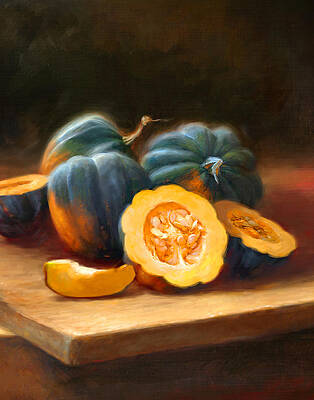The artwork is a detailed watercolor painting of a kitchen scene. The composition features a dark background, painted in deep shades of black and brown, which contrasts sharply with the brightly lit foreground. Central to the scene is a light wooden table or cutting board, upon which an array of acorn squashes is displayed. Three entire, uncut squashes, characterized by their dark green and orange-hued skins, are prominently positioned in the middle. In the foreground, a few squashes are sliced open, revealing their vibrant orange interiors filled with seeds. One large, bisected squash sits alongside another, and there is a small sliver showing more of their internal texture. Further back, an additional squash half is visible, highlighted by its distinct shape and color. The overall composition captures the rich, textural contrast between the wooden surface and the organic forms of the squash, giving a sense of both still life and culinary preparation.